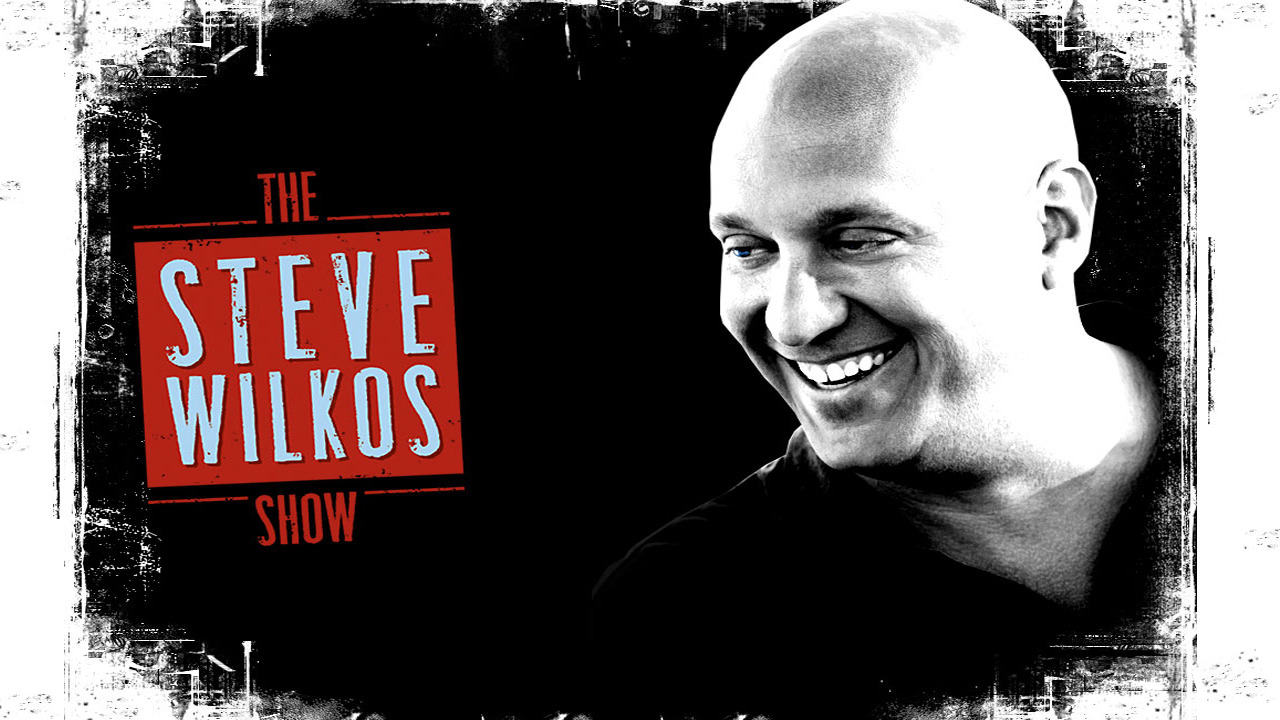This image is a promotional bumper for "The Steve Wilkos Show." On the right side of the image, Steve Wilkos, the well-known actor and bouncer, is featured prominently. He is smiling gently with his eyes glancing downward, showcasing his distinctive bald head. Steve is wearing a dark polo shirt that seamlessly blends into the black background, creating a dramatic and cohesive look. The image appears heavily edited, adopting a striking black and white theme. The only splash of color is the show's logo, situated in the center-left. The logo reads "THE" in red letters, followed by "Steve Wilkos" displayed in a light-colored font within a red rectangular box. Below this box, the word "SHOW" is also in red letters. The entire background is characterized by a stylishly torn black effect, with white elements giving it a dynamic, spear-like appearance, enhancing the image’s overall edgy and intense atmosphere.